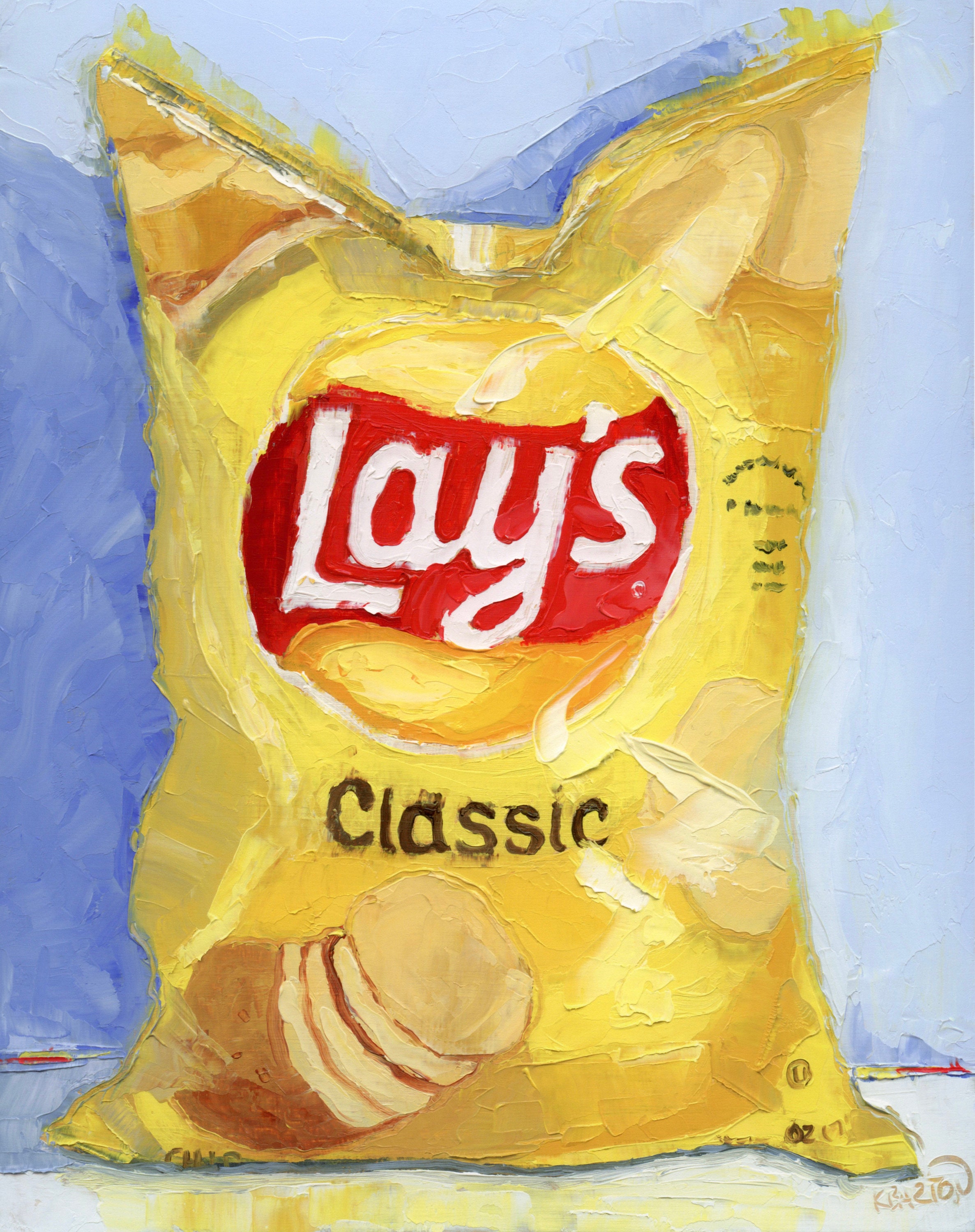This detailed painting depicts a large, classic-style Lays potato chip bag, rendered with oil paints on canvas. The bag, predominantly yellow with gold and orange hues, stands upright against a light blue background, which transitions to a darker blue shadow on the left side, creating depth and dimension. At its base, there's a subtle reflection, suggesting it might be standing on a reflective surface. The bag features a prominent white circle in the center, framed by a yellow sunburst design with a red banner bearing the iconic "Lays" logo in white lettering. Below this, the word "Classic" appears in black text. The bag also showcases an image of a potato sliced into chips, situated beneath the branding. Additionally, there are some illegible green words on the right side of the bag. The artist's signature, messy and smudgy, is located in the lower right corner of the painting. The overall composition emphasizes the bag, with the contours captured through varied colors rather than clean lines, giving it a slightly abstract, textured appearance.